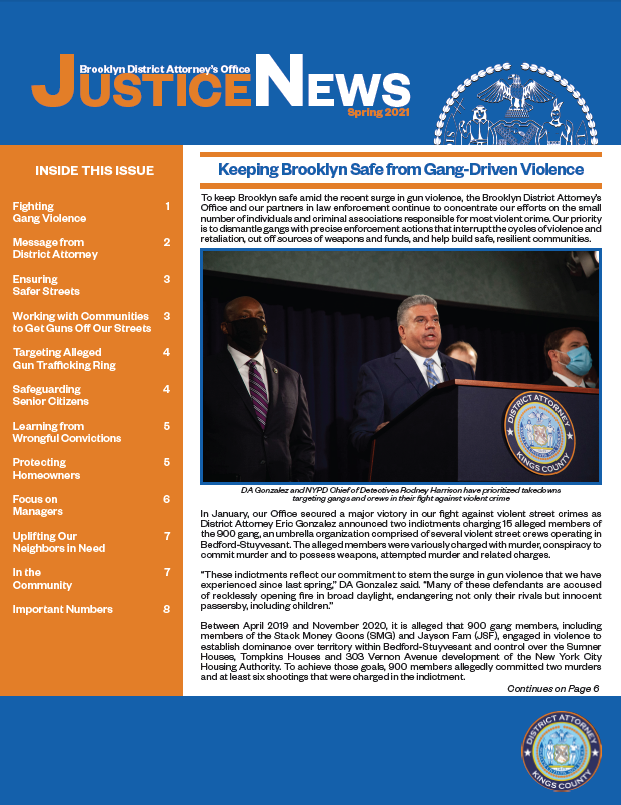This image is the newsletter cover for the Brooklyn District Attorney's Office titled "Justice News." The top of the image features a blue background with a white text that reads "Brooklyn District Attorney's Office" followed by "Justice" in orange and "News" in white. Below "News," the issue date "Spring 21" is highlighted in orange. On the right side of the header, there is a white logo.

Running down the left side is an orange column listing the sections included in this issue. These sections are: 
1. Fighting Gang Violence
2. Message from the District Attorney
3. Ensuring Safer Streets
4. Working with Communities to Get Guns off Our Streets
5. Safeguarding Senior Citizens
6. Learning from Wrongful Convictions
7. Protecting Homeowners from Fraud
8. Focus on Managers
9. Uplifting Our Neighbors in Need
10. Important Numbers

To the right of this list, the headline "Keeping Brooklyn Safe from Gang-Driven Violence" introduces the main article.